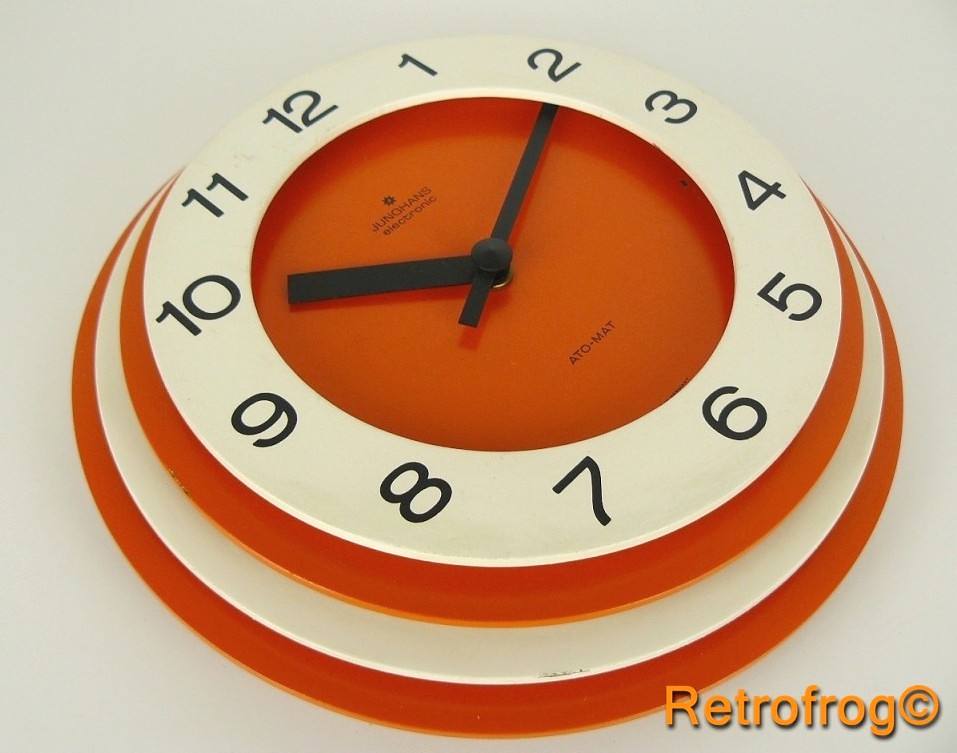This photograph features a vintage-inspired clock reminiscent of the 1960s or 1970s design aesthetics. The clock is composed of a visually appealing stack of concentric circles, each boasting its own distinct coloration. The base and widest part of the clock is a rich, deep reddish-orange circle. Moving inward, the next ring is a creamy beige-white color, followed by a smaller orange circle. At the center lies the main clock face, a pristine white circle adorned with numerals around its edge, encased by another orange ring on the inside. The time displayed on the clock is approximately 10:10. In the bottom-right corner of the image, the text "Retro Frog ©" is subtly inscribed, adding a touch of authenticity to the retro vibe.